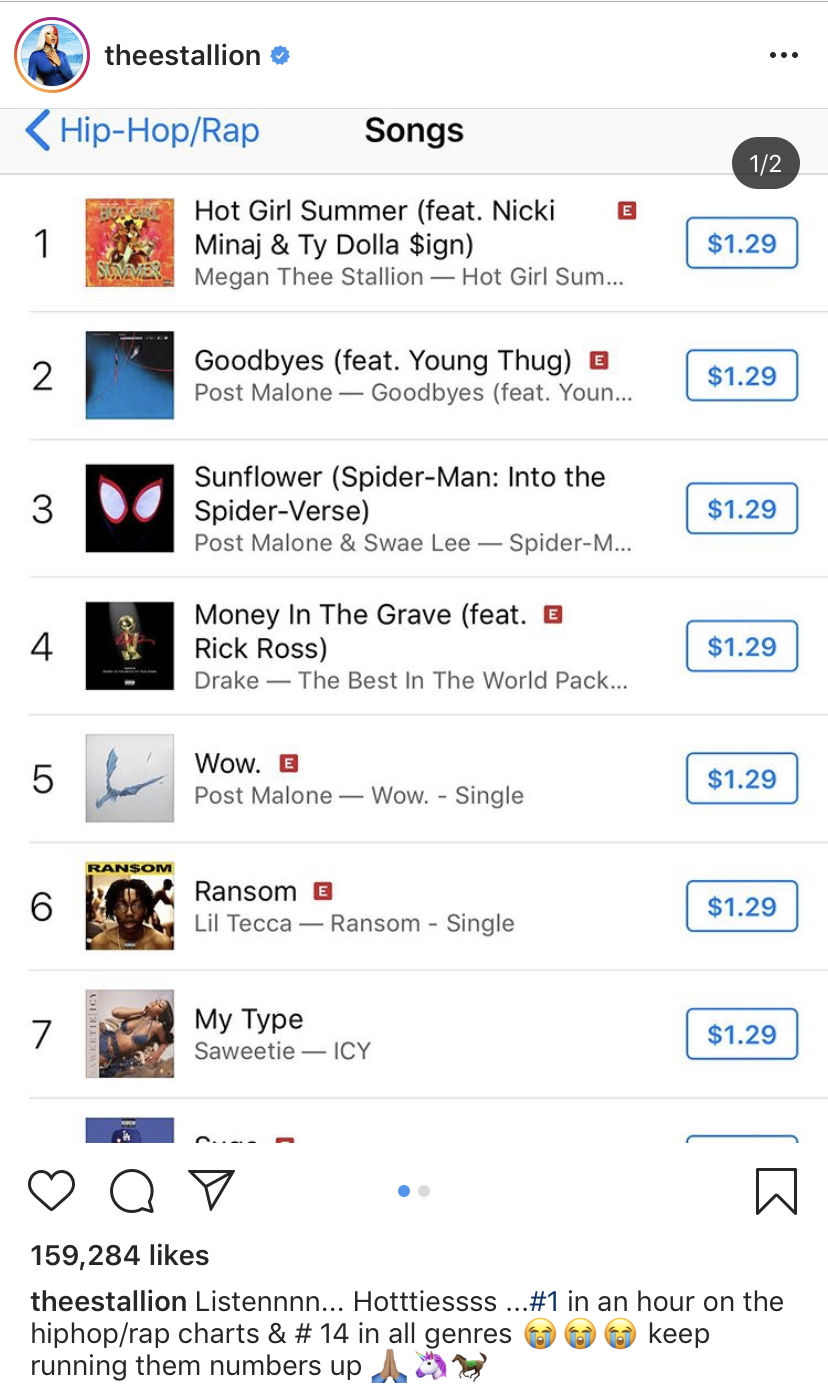The image showcases a music playlist from a mobile device featuring various hip-hop and rap songs. In the upper left corner, there is a circular icon depicting a female figure against a blue sky backdrop, identified as "The Stallion" with a verified checkmark beside her name. Adjacent to this, in the top right corner, are three vertical dots indicating more options. The header is highlighted in blue and categorizes the genre as "Hip-Hop/Rap Songs."

The playlist displays seven songs:

1. **Hot Girl Summer** (featuring Nicki Minaj and Ty Dolla $ign) - Priced at $1.29
2. **Goodbyes** (featuring Young Thug) - Priced at $1.29 with a purchase button beside it.
3. **Sunflower** (from *Spider-Man: Into the Spider-Verse*) - Priced at $1.29
4. **Money in the Grave** (featuring Rick Ross) - Priced at $1.29
5. **Wow** by Post Malone - Priced at $1.29
6. **Ransom** by Lil Tecca - Priced at $1.29
7. **My Type** by Saweetie (labeled here as Saw Weedy) - Priced at $1.29

At the bottom of the screen, there are interactive icons including a heart, a conversation bubble, and a paper airplane. The post has gathered 159,280 likes. Below this are details from The Stallion, stating: "Listen, Hottiness, number one in an hour on the hip-hop rap charts and number 14 in all genres,” followed by three smiling emojis. The caption encourages fans to continue streaming with the phrase "keep running them numbers up," and concludes with prayer hands, unicorn, and horse emojis.